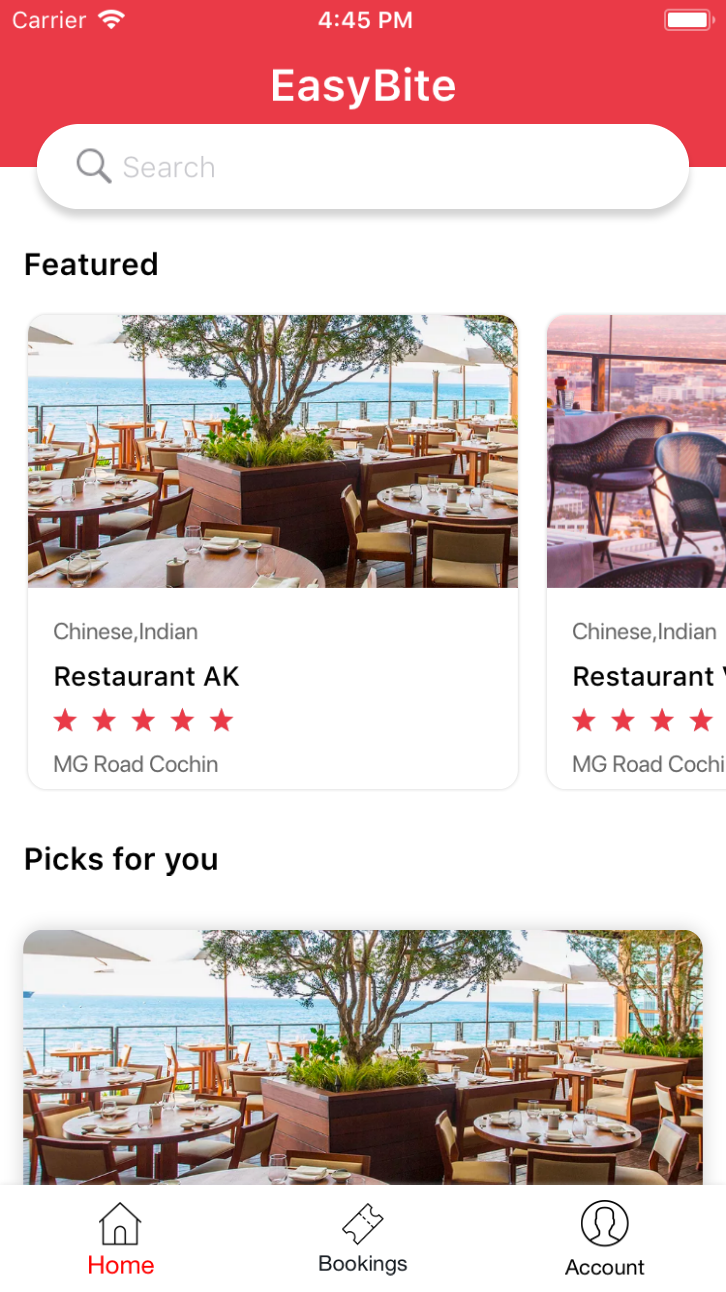**Detailed Caption:**

This image is a screenshot from a mobile app. In the top-left corner, the word "carrier" is displayed in white text, accompanied by a white Wi-Fi symbol. The current time, "4:45 p.m.," is indicated at the center top, with a white battery icon on the top-right corner.

Beneath this, in larger white text, the app's name "Easy Bite" is prominently displayed. Below the app name is a search bar with the placeholder text "Search" and a small magnifying glass icon. 

The main content features a section labeled "Featured" in black text. This section showcases a thumbnail image of a dining area with multiple tables adorned with various plates and drinks. The tables are centered around a plant with a small tree, and a bay area is visible in the background, adding to the ambiance.

Underneath the thumbnail, the text lists "Chinese" and "Indian" cuisines followed by "Restaurant A.K." accompanied by a rating of five red stars. Below this, the location "MG Road, Kachin" is written in gray text.

To the right of this information is another partially visible image showing a couple of chairs and a cityscape in the background, suggesting an evening setting. The text "Restaurant" is visible but cut off, and there are additional stars indicating a rating.

Below this section, another label, "Pics for You," is displayed, featuring the same dining area image with the bay area background.

At the bottom of the screen, the navigation options "Home," "Bookings," and "Account" are clearly shown, providing easy access to different sections of the app.